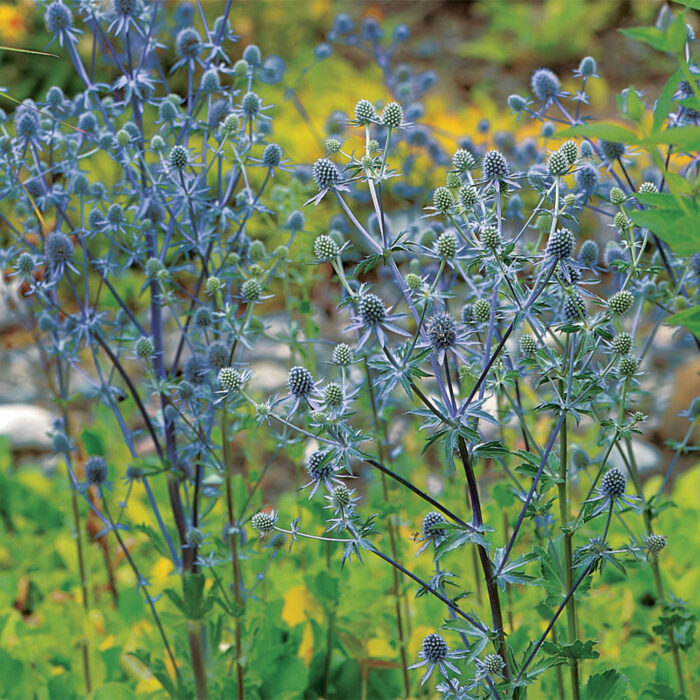In the foreground of the image stands a plant that closely resembles a thistle, with striking blue-gray foliage and underdeveloped flower buds at the top of each stem. The plant is somewhat dried, exhibiting silvery, almost light gray tones with sparse leaves concentrated around the budding areas. The background is an out-of-focus expanse of lush green foliage, with hints of yellow and brown, adding a soft contrast and an indication of a thriving, wild habitat. The surrounding greenery, both beneath and behind the featured plant, provides a vibrant and slightly blurred backdrop, ensuring that all attention is drawn to the unique, almost ethereal quality of the blue-gray thistle-like plant in sharp focus.